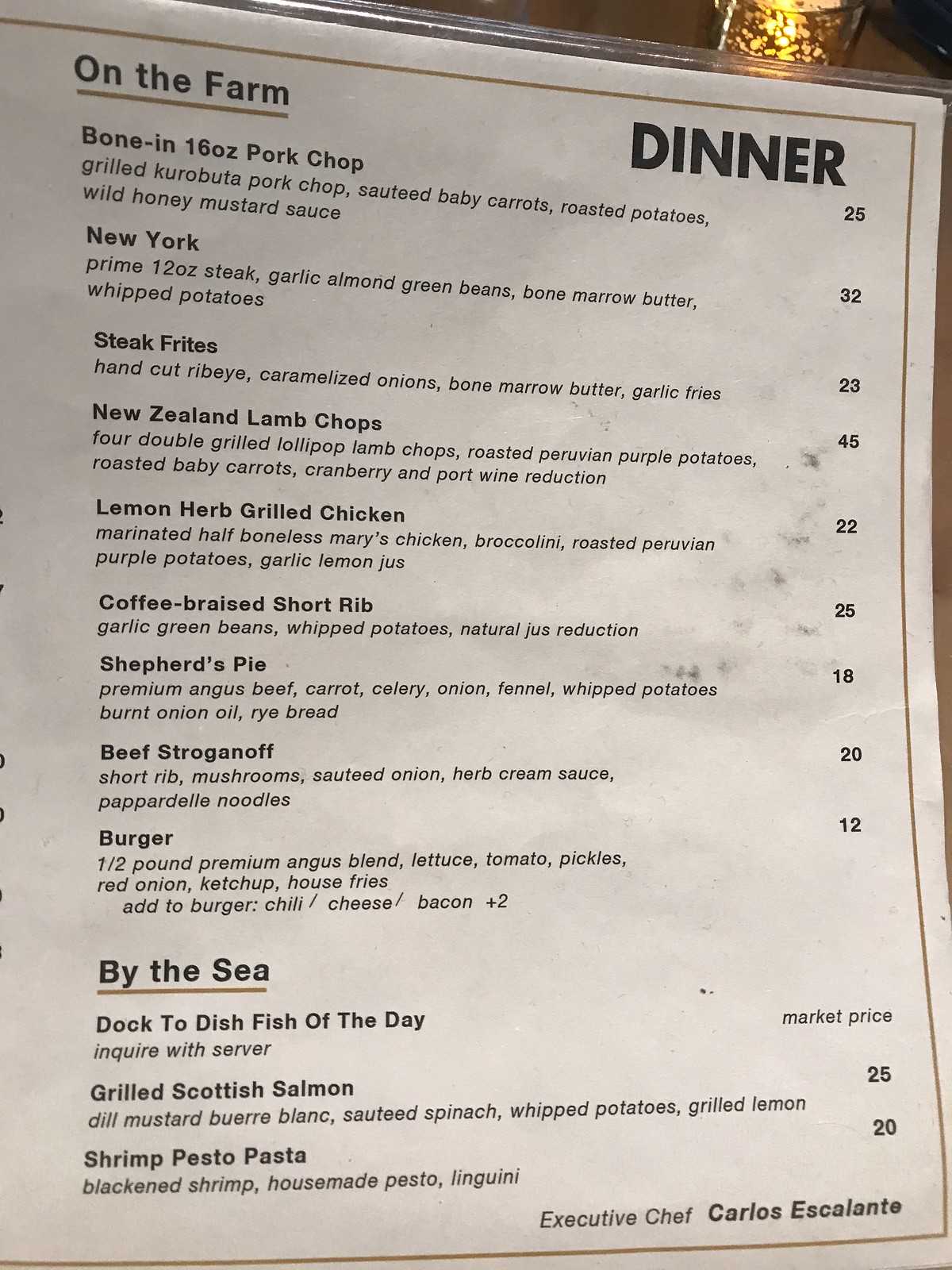The image captures a rustic dining scene with a partially held up menu in the foreground. The menu, a white sheet of paper protected by a silver wrapper, features a golden border. It prominently displays "DINNER" in black capital letters at the top right corner, and "ON THE FARM," underlined in gold, to the left. Behind the menu, a brown, ornate candle holder with a burning yellow flame adds to the warm, rustic atmosphere.

The menu lists an array of delectable dishes:

1. **Bone-in 16-ounce Pork Chop**: Grilled Currubata pork chops, sautéed baby carrots, roasted potatoes, wild honey mustard sauce. - $25
2. **New York Steak**: Prime 12-ounce steak, garlic almond green beans, bone marrow butter, whipped potatoes. - $32
3. **Steak Frites**: Hand-cut ribeye, caramelized onions, bone marrow butter, garlic fries. - $23
4. **New Zealand Lamb Chops**: Four double grilled lollipop lamb chops, roasted Peruvian purple potatoes, roasted baby carrots, cranberry and port wine reduction. - $45
5. **Lemon Grilled or Herb Grilled Chicken**: Marinated half boneless Mary's chicken, broccolini, roasted Peruvian purple potatoes, lemon garlic juice. - $22
6. **Coffee Braised Short Rib**: Garlic green beans with potatoes, natural juice reduction. - $25
7. **Shepherd's Pie**: Premium Angus beef, carrot, celery, onion, fennel with potatoes, burnt onion oil, rye bread. - $18
8. **Beef Stroganoff**: Short ribs, mushrooms, sautéed onions, herb cream sauce, pappardelle noodles. - $20
9. **Burger**: Half pound of premium Angus blend, lettuce, tomato, pickles, red onion, ketchup, house rice. Add chili, cheese, bacon for an additional $2. - $12

**By the Sea** options include:
- Fish of the Day
- Grilled Scottish Salmon
- Shrimp Pesto Pasta